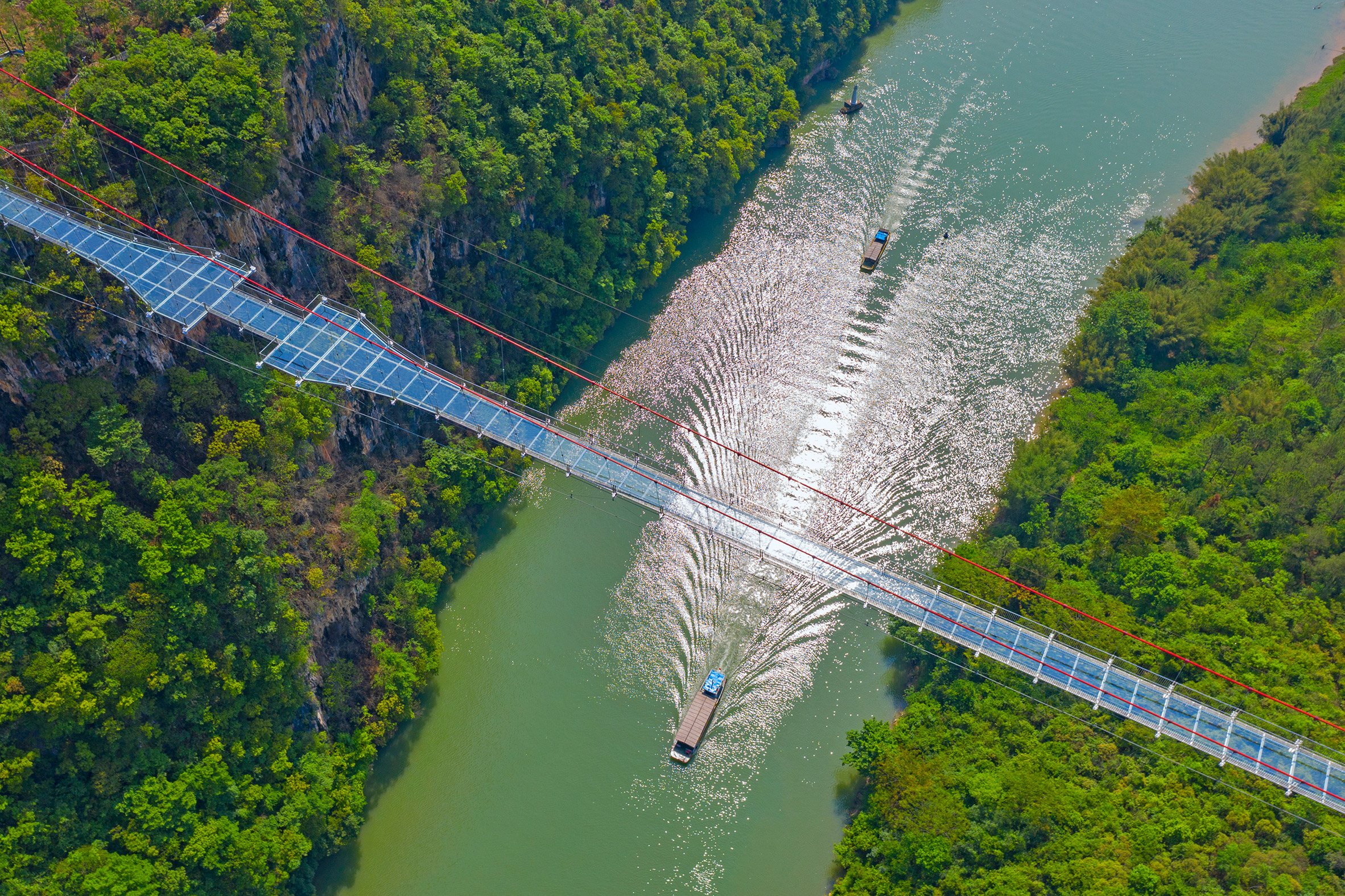This bird's-eye view photograph captures a serene scene of a large, lush green canal flanked by dense forest on both sides. The water in the canal is a striking green, reflecting the bright daytime sunlight. A significant detail is the high bridge spanning the canal, resembling a geometric network of blue squares and thin white wires. The bridge doesn't appear to be a standard concrete structure; rather, it looks more like it's made of delicate red string and a gray path, invoking a sense of fragility. Beneath the bridge, a large boat navigates the canal, trailed by a smaller boat, both leaving visible streams in the water from their propulsion. On the left side of the canal, you can see a cliffside, adding to the dramatic landscape. A buoy can also be spotted near the boats, enhancing the detail of this vivid, nature-filled scene.